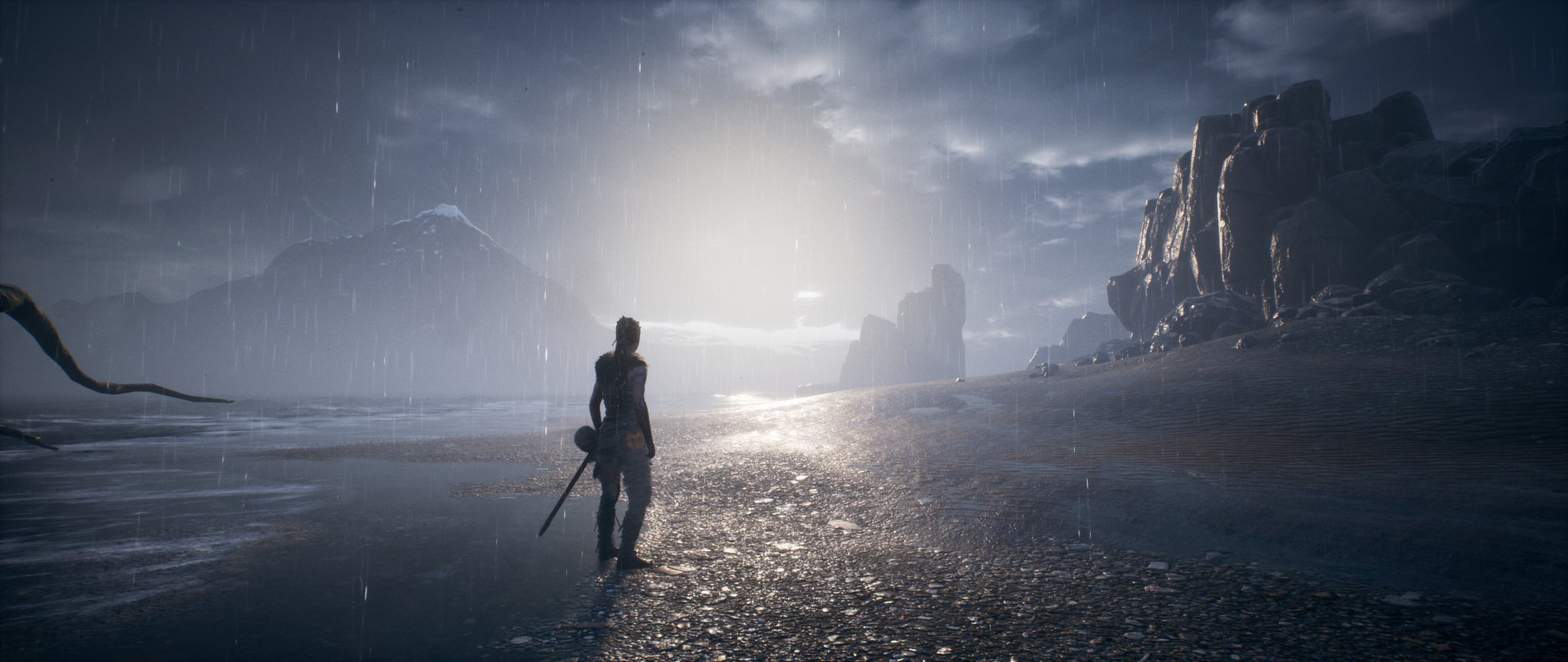This detailed image, seemingly a computer-generated screenshot from the video game "Hellblade: Senua's Sacrifice", showcases a somber, coastal landscape. The scene features a character resembling a Viking woman, standing on a pebbled stone beach with the water from the ocean lapping in from the bottom left corner. She is clad in light gray armor over her torso and legs, with dark shoes, and has short hair tied into a ponytail. A sheathed sword hangs on her left side.

The backdrop includes a rugged beach, slightly inclined, leading to a rocky structure on the top right. In the far distance to the left, a snow-capped mountain rises against a dark blue sky scattered with clouds. The sky varies from thick, dark gray clouds interspersed with some blue and white, to a radiant light source in the center, casting reflections on the wet, rock-strewn ground.

Additional elements include rough, grayish-blue water with white caps and puddles on the right side, a large cliff exhibiting shades of brown and gray, and distant mountain ranges both left and right of the central light. A dim sun peeks through the clouds, casting a soft beam of light while green rain falls around the character, enhancing the scene's mysterious and atmospheric tone.